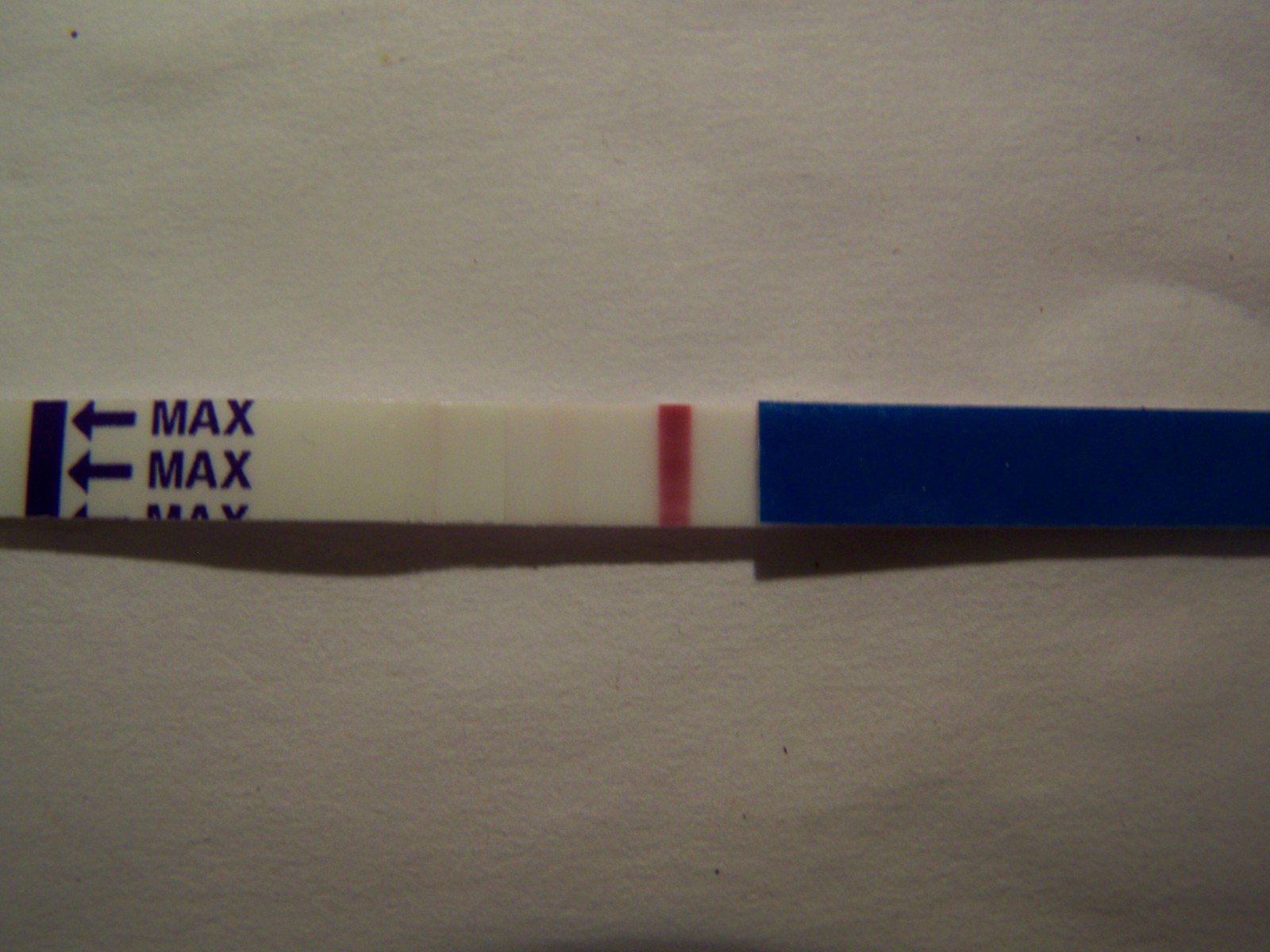The image features a textured, light gray background, possibly made of paper or cloth, displaying subtle wrinkles and small puffs throughout. A faint semi-circle imprint is noticeable within the fabric. Centrally positioned, there is a long plastic stick, which appears to be a test strip. The lower half of the strip is dark blue, transitioning into a white section adorned with a single red stripe just above the blue area. The upper part of the stick is predominantly white, bearing the word "MAX" repeated three times in blue letters. To the immediate left of "MAX," three blue arrows point towards a prominent blue line that runs vertically from the top to the bottom of the stick. Additionally, the shadow of the dipstick is visible along one side, casting a slight contrast against the textured background. The overall scene suggests this item could be a pregnancy test or a similar type of dip test.